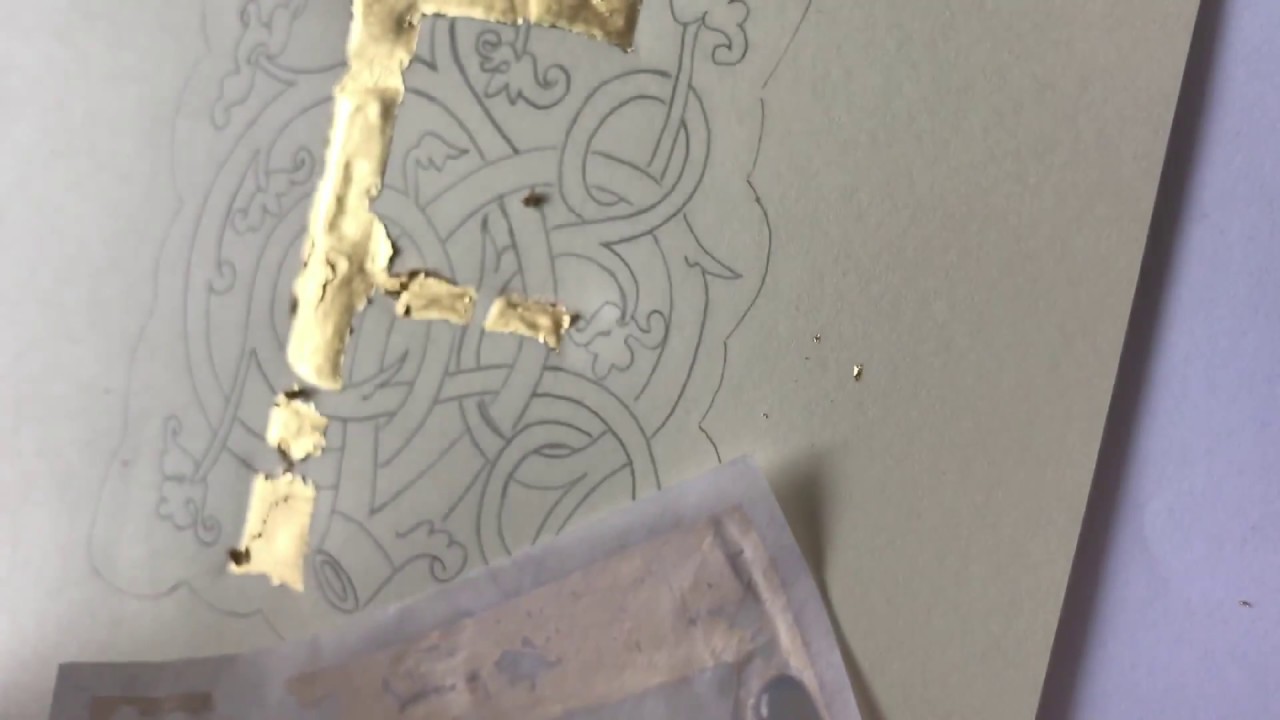The image depicts a highly detailed pencil drawing on what appears to be a piece of quality cardstock or watercolor paper. The drawing features intricate swirls and looping lines, reminiscent of delicate calligraphy or perhaps a decorative crest. Superimposed over the drawing is a gold foil 'F', although it seems to be partially incomplete or haphazardly applied. The 'F' does not seamlessly integrate with the pencil work, suggesting it might be an unfinished monogram, possibly with some remaining gold foil dust to be cleaned up. The image also shows another piece of slightly transparent paper beneath the main drawing, likely transfer paper for the gold leaf. The setting includes a bluish-gray background, and the papers appear to be lying on a rough, perhaps wrinkled surface that hints at some fabric or cloth beneath. There's a small smudge between the top and bottom of the 'F' that disrupts the otherwise formal appearance of the work.